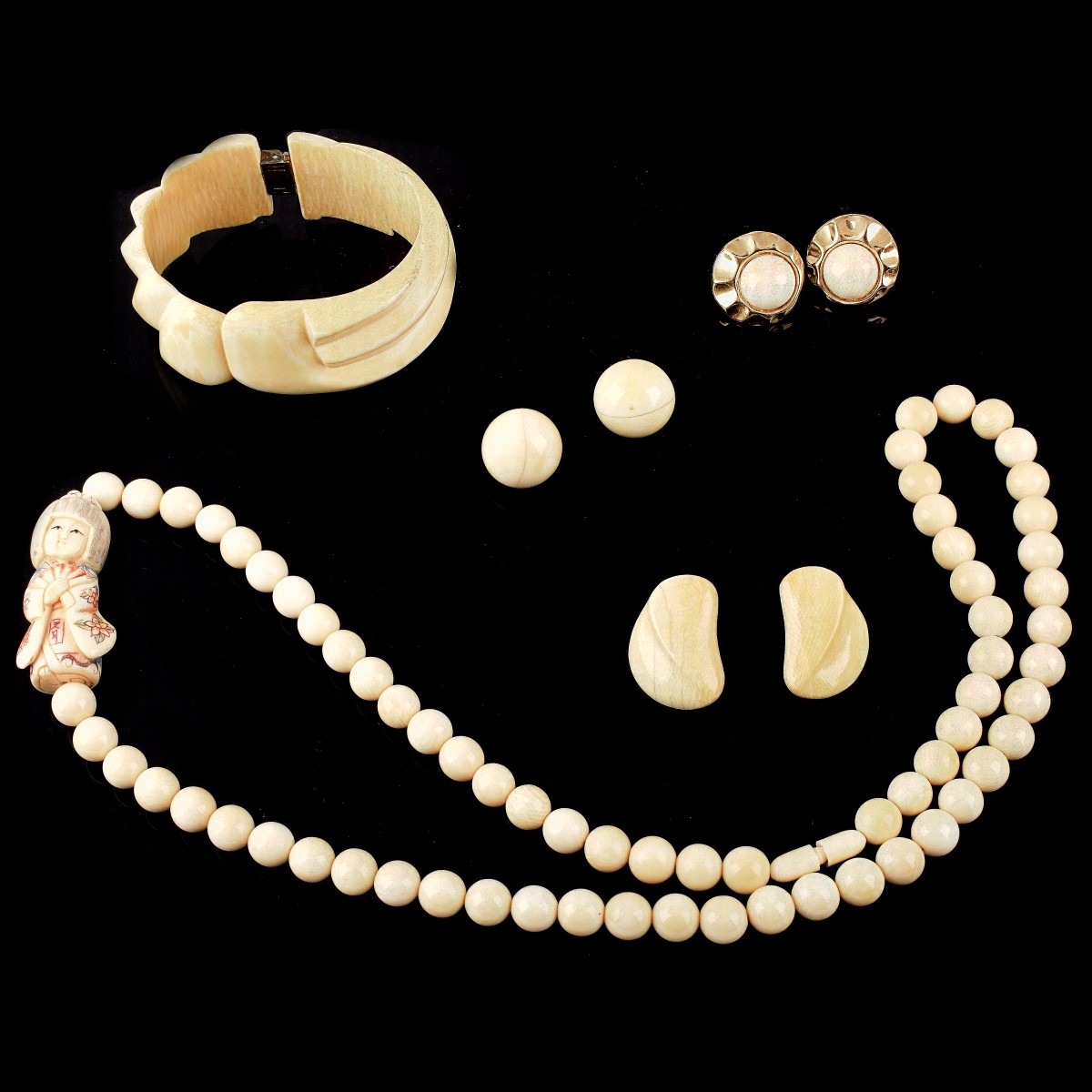The image features an assortment of jewelry displayed against a pitch-black, velvety background, which makes the white and gold elements stand out vividly. Central to the composition is a white pearl necklace, artistically arranged in a gentle curve resembling a smile. At the heart of the necklace is a small, intricate statue of a Japanese woman adorned in a traditional kimono, adding a touch of cultural elegance. Surrounding the necklace are three distinct pairs of earrings: one pair is purely white and circular, another pair features circular white pearls encircled by gold, creating a flower-like appearance, and the third pair has an oblong shape in white. Additionally, a sophisticated white bracelet, designed to open and close over the wrist with ease, is positioned above the necklace, complementing the ensemble. Together, these pieces create a striking and harmonious display, highlighted by the black background which enhances the visual impact of the white and gold jewelry.